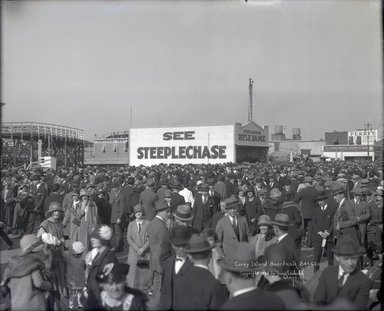This black and white photo, dating from the early 1920s, captures an outdoor scene densely packed with thousands of people. Men, dressed in suits, ties, and long trench coats, and women, adorned in dresses and round hats, fill the space. The crowd's attire reflects the era's fashion, with men sporting Derby-style hats. In the background stands a large building with a triangular facade, possibly resembling a warehouse. A prominent sign on its white wall reads, "See the Steeplechase." There is also a tall structure behind the building, likely a radio tower. To the far left, a pier or wooden roller coaster is visible, suggesting this gathering might be part of a fair or an amusement park event. The image portrays a bustling scene of early 20th-century public life, with rows of people awaiting their turn to enter what appears to be a newly-opened stadium, marking an eventful day replete with excitement and confusion over seating arrangements.